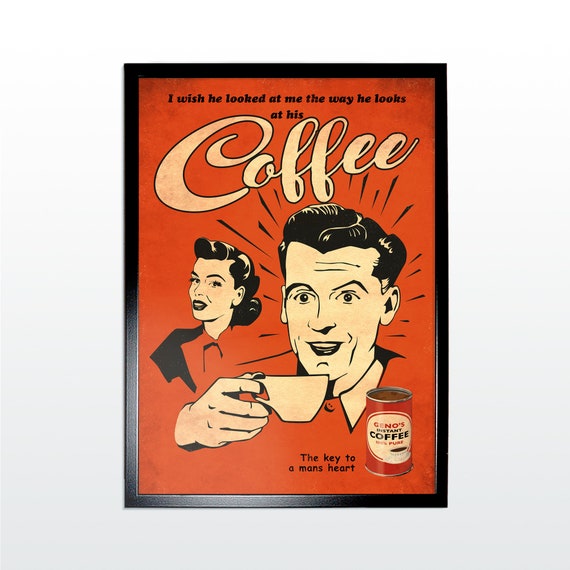This framed advertisement poster from the 1940s or 50s features a striking red background with a black border. Central to the image is a vintage, cartoon-style illustration of a man and a woman. The man, located on the right side of the poster, has black hair and is depicted holding a coffee mug in his right hand, his expression one of sheer delight, emphasized by white, wide-open eyes and radiating lines around his head. To his left, a woman, also with black hair and dark lipstick, gazes at him, seemingly pleased with his reaction. Both figures are dressed in red that blends into the backdrop.

At the top of the poster, bold black text reads, "I wish he looked at me the way he looks at his." Below this, in large, curvy light tan font, is the word "coffee." At the bottom right corner of the image, a small can of coffee labeled "Gino's," though the specific details are unclear, is accompanied by the slogan, "the key to a man's heart," reinforcing the theme that a delicious cup of coffee holds a special place in the man's affections. The overall aesthetic and color scheme draw attention to the nostalgic charm of the advertisement, capturing the viewer's eye with its vivid contrasts and humorous sentiment.